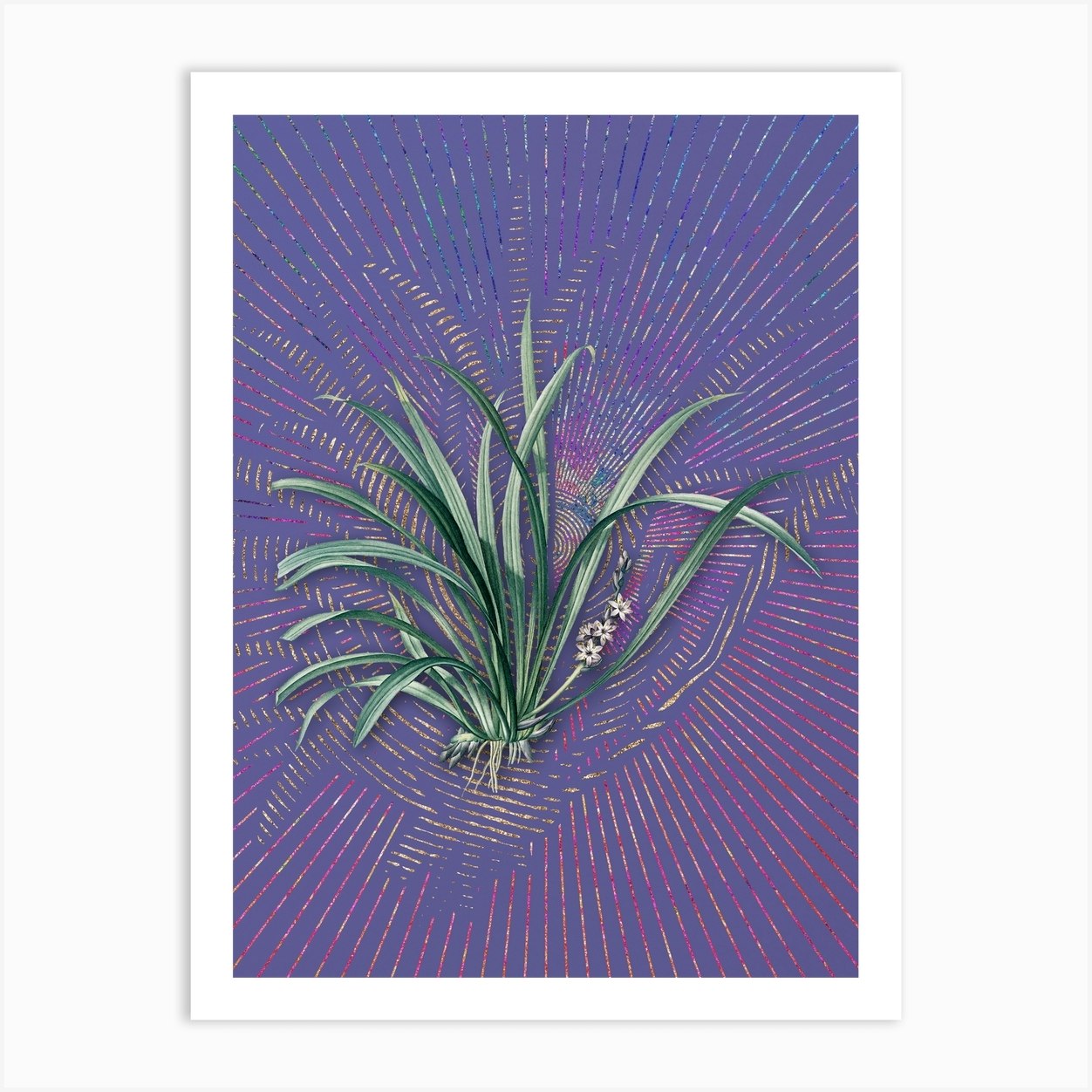The image showcases a whimsical and vibrant artwork set against a dynamic, predominantly purple background that is far from solid, as it features swirling lines and intricate patterns in various colors such as yellows, pinks, reds, blues, and greens. At the center of the image, a striking green plant with long, sprawling leaves commands attention. The plant is depicted with visible white roots and is adorned with starburst-like white flowers. The whimsical design includes both circular and straight lines, creating an enchanting, almost ethereal effect. This artistically made piece, with its detailed and colorful composition, would be a delightful addition to a hotel or a plant lover's home. The photograph is matted with a white border, further enhancing the overall presentation of this captivating artwork.